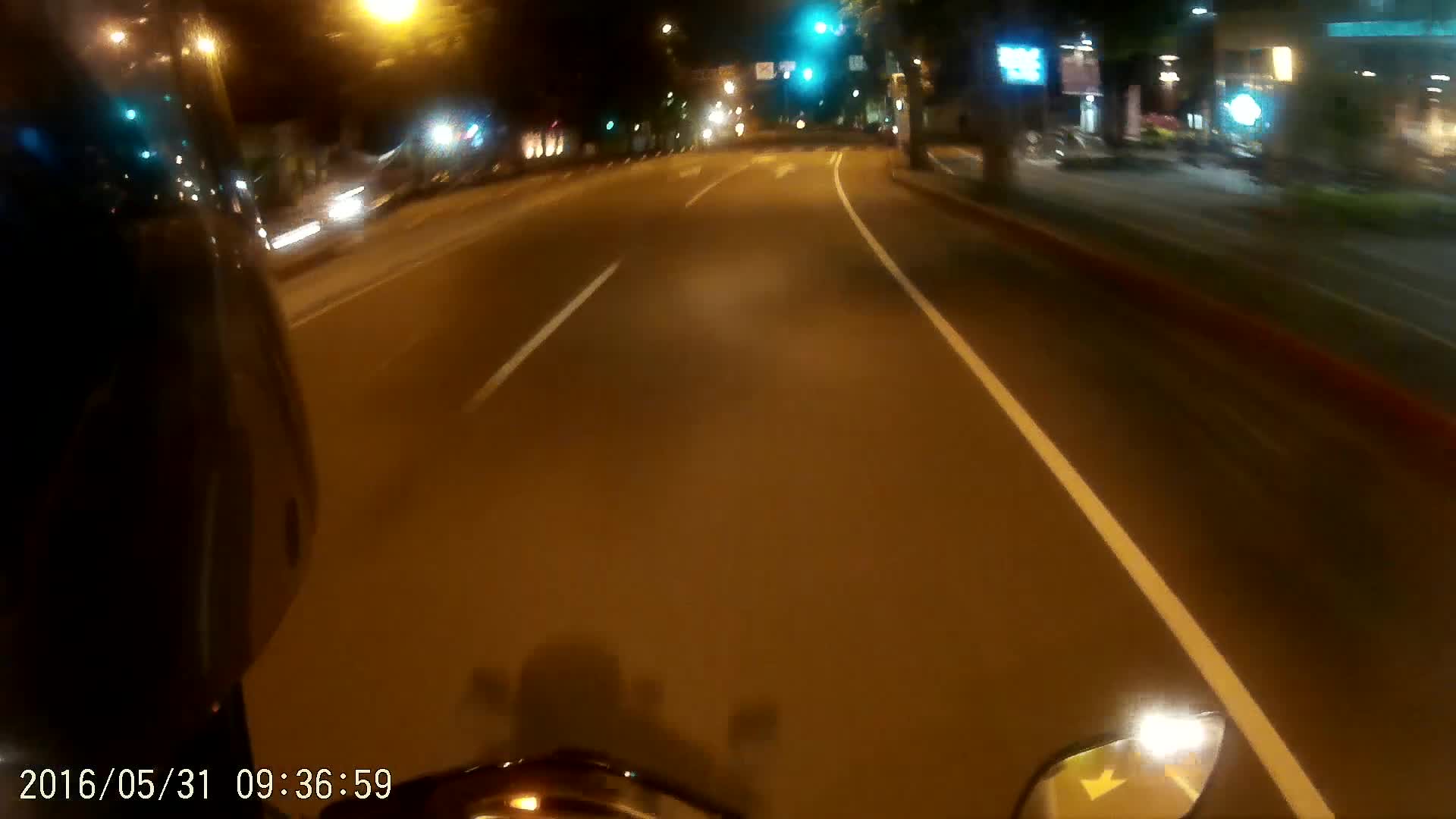This color photograph, taken at night in a city setting, offers a motorcyclist's perspective of a two-lane roadway. The image seems captured from either a camera mounted on the motorcycle or by a passenger sitting at the rear. In the foreground, the motorcyclist's black helmet is visible on the left side, along with the center cowl and the right-side rearview mirror at the lower edge, bearing an arrow pointing down. The asphalt road stretches ahead with a solid white line on the left and a dashed line in the middle, flanked by blue and yellow street lights on each side. The dark black sky contrasts with the various lights illuminating the area, including street lights and green traffic lights further down the road. Lit-up buildings, including storefronts with lots of glass, can be seen on the right and left, though they appear slightly blurry and out of focus. The roadway is devoid of other vehicles, and the motorcyclist's shadow is cast onto the street. The image is timestamped in the lower left corner with the date "2-16-05-31" and time "0-9-36-59."